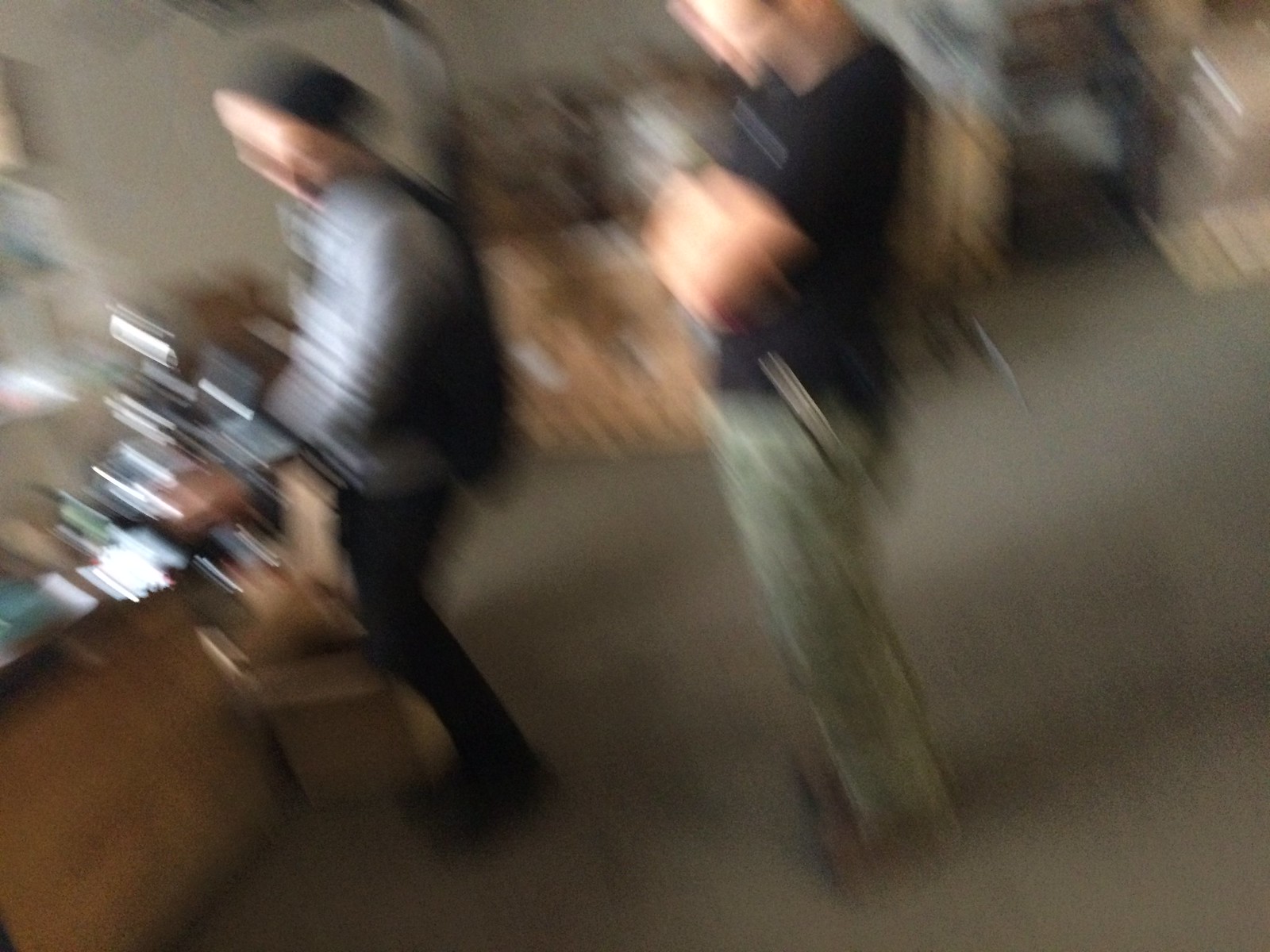An indistinct, blurry photograph depicts a scene indoors with gray carpeted flooring. On the left side of the image stands a table, partially visible. In front of the table, a person is captured wearing a shirt, a black vest, and black pants. Their hands are extended forward, possibly in the act of making or placing something, although the object in their hand remains unclear due to the blur. Illuminated by a light source that highlights their face, they draw attention within the scene. Beside them, another individual with a black shirt and green pants, looks downward. The background features mostly brown hues and white walls, adding an impressionistic backdrop to the scene.